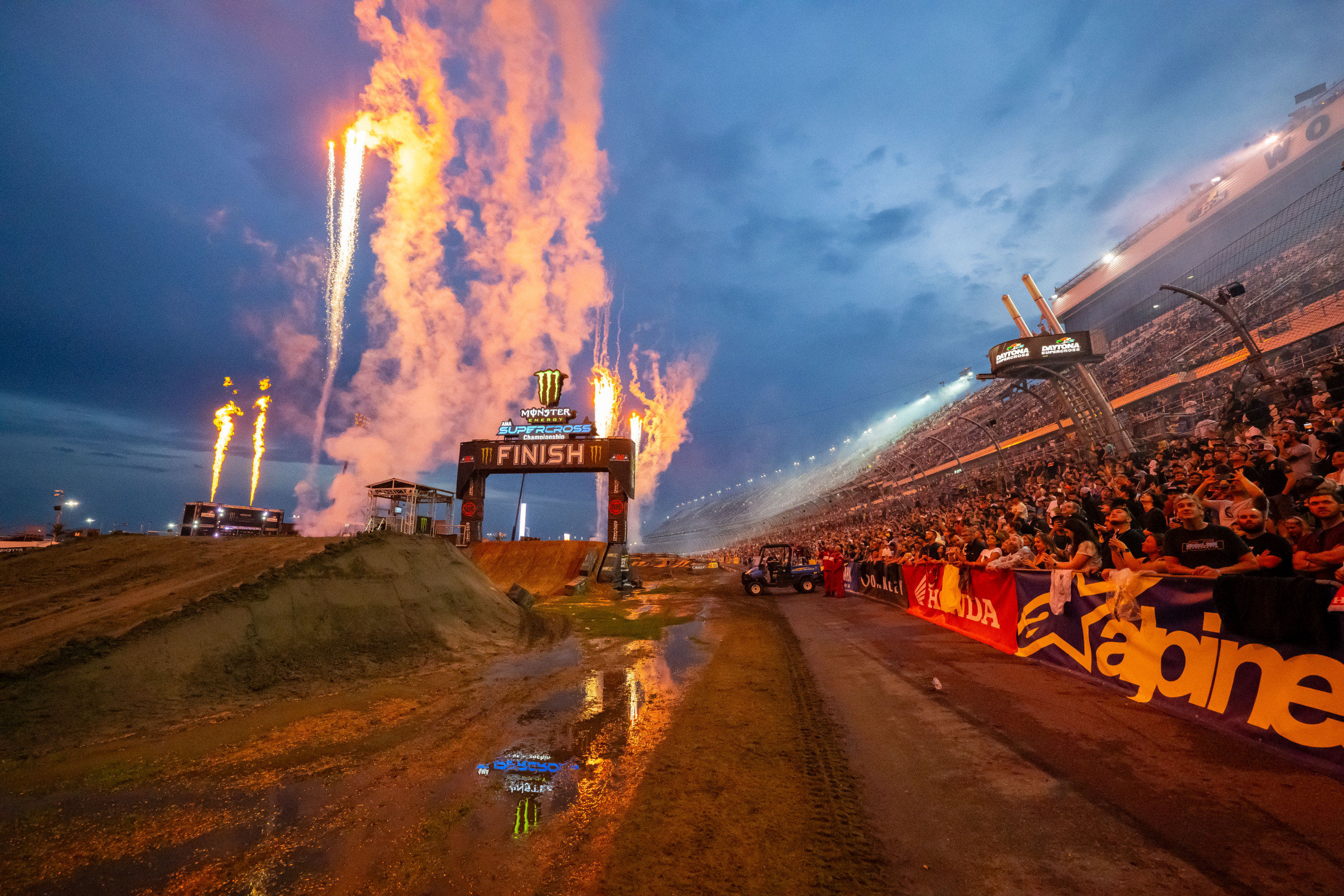The image captures a thrilling moment at a professional Super Motocross Championship event during the twilight hours, just as the sky transitions from dusk to dark. The expansive view showcases the clayish red dirt track with its inclines and challenging hills, designed for intense racing conditions. Prominently featured is the illuminated "Supercross" finish line adorned with neon lights, above which vibrant fireworks explode, casting a radiant pink smoke and flames into the sky.

The grandstands on the right are packed with eager fans, their presence slightly muted yet palpable, cheering enthusiastically as the race unfolds. Along the seats, eye-catching sponsor banners from well-known brands like Alpine and Honda add splashes of yellow and red. Further details include a couple of indistinct vehicles in the background, possibly safety carts, and the murky presence of water and mud splattered across the track, heightening the sense of a high-energy, action-packed atmosphere. The overall scene is bathed in the colorful glow of varied light sources, creating a mesmerizing backdrop for this adrenaline-fueled sporting event.